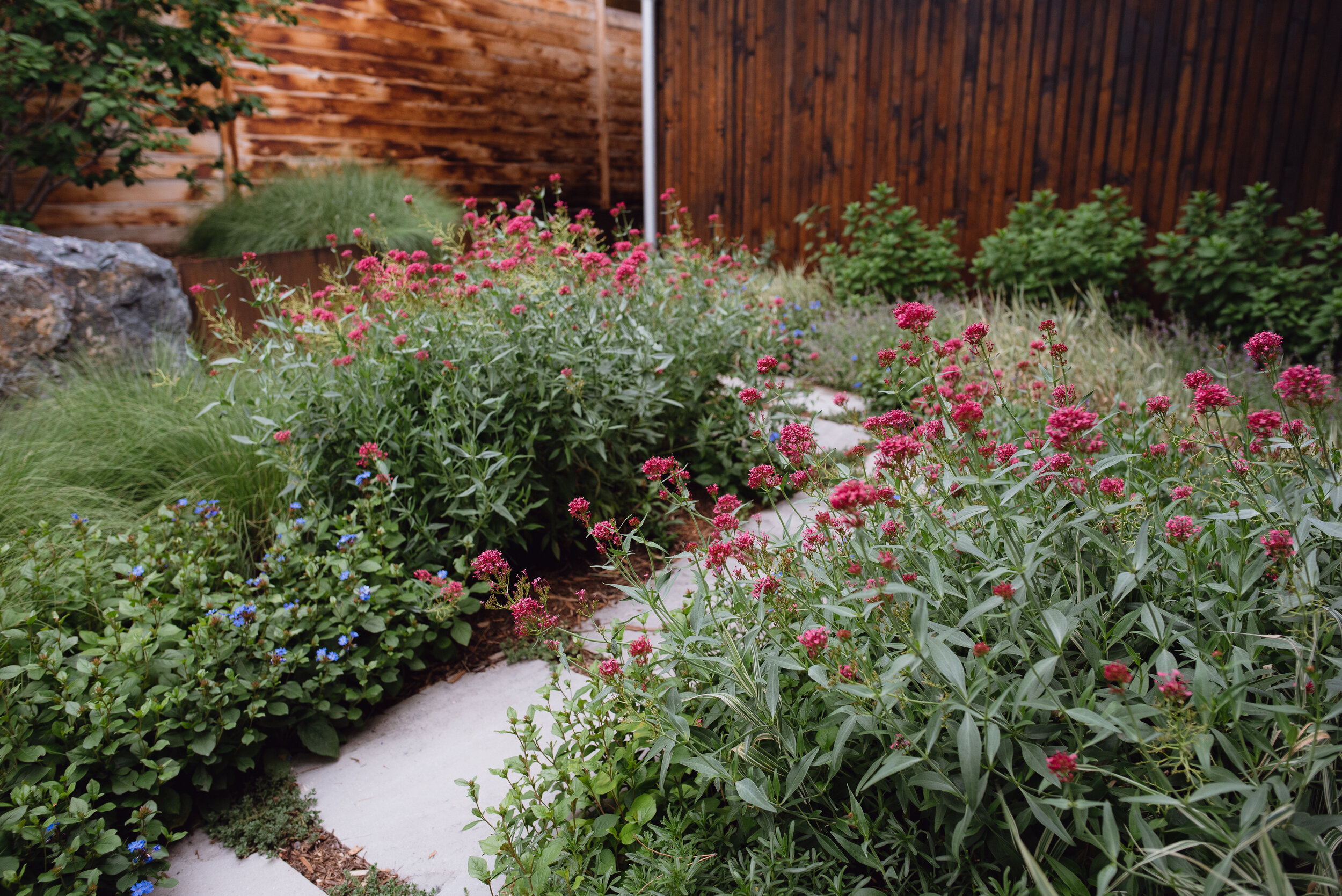The image depicts a landscaped backyard walkway framed by verdant plant life and vibrant blossoms. The setting appears to be behind a wooden house with wood slat siding and a rich brown wood slat fence. A white, irregular-shaped stone pathway meanders from the bottom left corner of the image, curving back toward the center before disappearing behind a cluster of tall flowering plants. On the left side of the path are plants bearing multiple red buds and blossoms, while the right side features lush green foliage and additional flowering plants with tall stems and red blossoms.

The backyard garden is a mix of green-leaved plants and colorful flowers, with a small gray boulder adding a natural touch to the scene. The colors in the photo prominently include greens from the plants, reds from the flowers, browns from the house siding and fence, and white from the stone pathway. The backdrop of the image shows a dark-stained wooden fence with vertical lumber pieces, and at its base are a few small green shrubs, contributing to the overall lush, serene atmosphere. In the far left, a red brick building adds an additional layer of texture and color, enhancing the realistic, representational style of this landscape photograph.